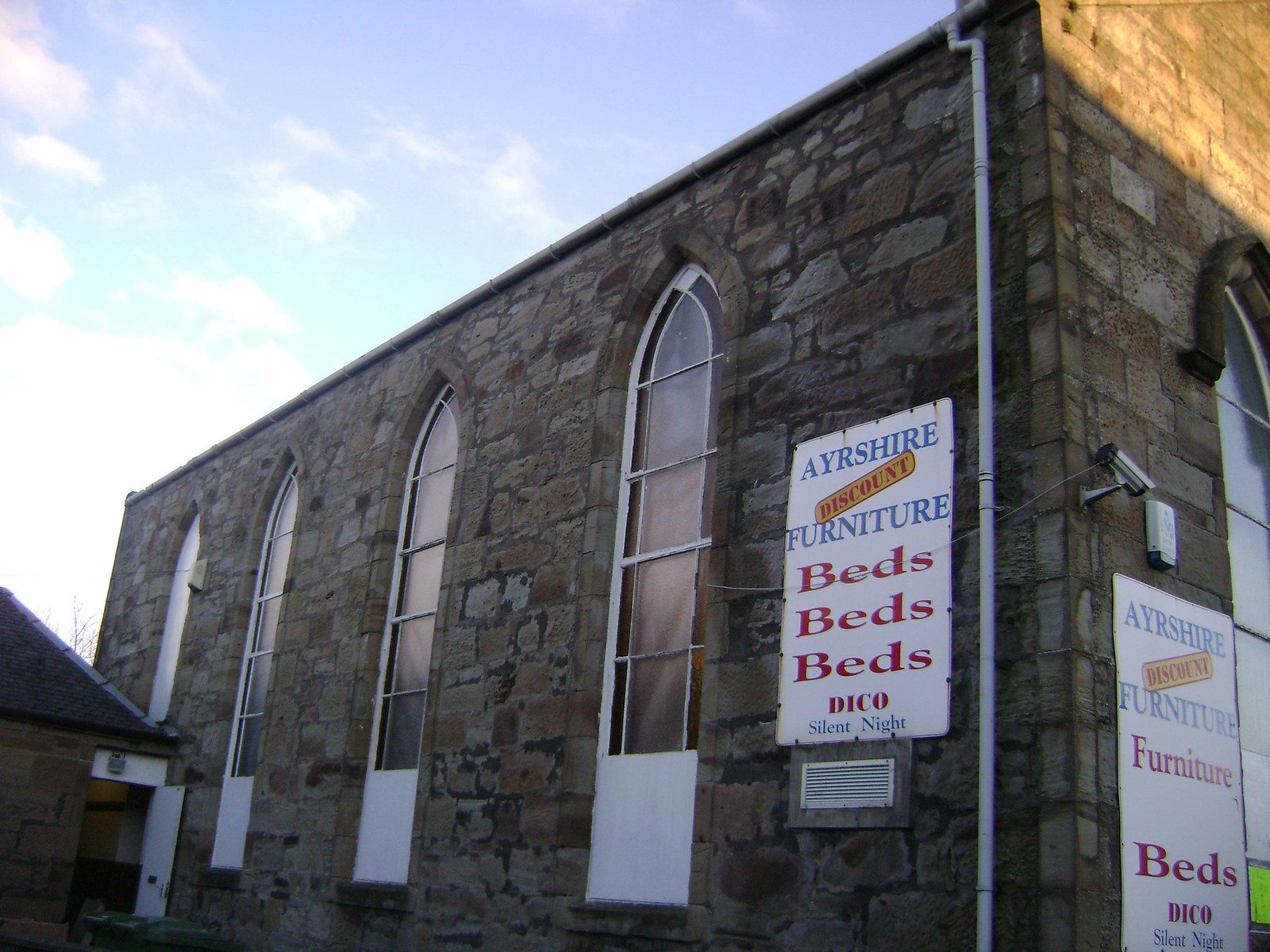The image depicts a large, old stone building constructed from interspersed beige and grayish stones. The corner of the building is prominently featured, with four arched windows running down the left side, their frames painted white. Various white signs with blue, red, and yellow lettering are attached to the building, advertising "Ayrshire Furniture," "Beds Beds Beds," and "Daiko." There is a notable vertical sign near one of the central windows that reads "Ayrshire Furniture" in blue text, with "DISCOUNT" stamped across it in yellow with red lettering, followed by "BEDS BEDS BEDS" in red and "DAIKO" and "SILENT NIGHT" in blue. The sky above is a light blue with streaks of turquoise closer to the building and soft, non-puffy clouds. A metal pipe runs down one side of the building, adding to its aged, rustic appearance.